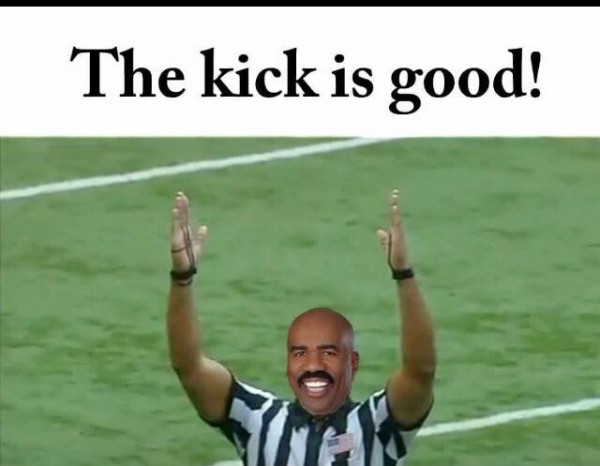The image features a humorous meme with a white background and a thick black line running horizontally across the top. Below the line, large black letters in a typewriter format exclaim, "THE KICK IS GOOD!" Above a color photograph. The photograph shows a green sports field, likely a football field, with two white lines running horizontally across it. In the foreground, a figure dressed as a referee is visible from the chest up, wearing a vertically striped black and white shirt with a faint American flag on the right side. The figure's arms are extended upwards in the "kick is good" signal, and the head has been superimposed with the smiling face of Steve Harvey, the well-known African American comedian. His bald head, big white teeth, and thick black mustache are clearly recognizable, adding a humorous twist to the image.